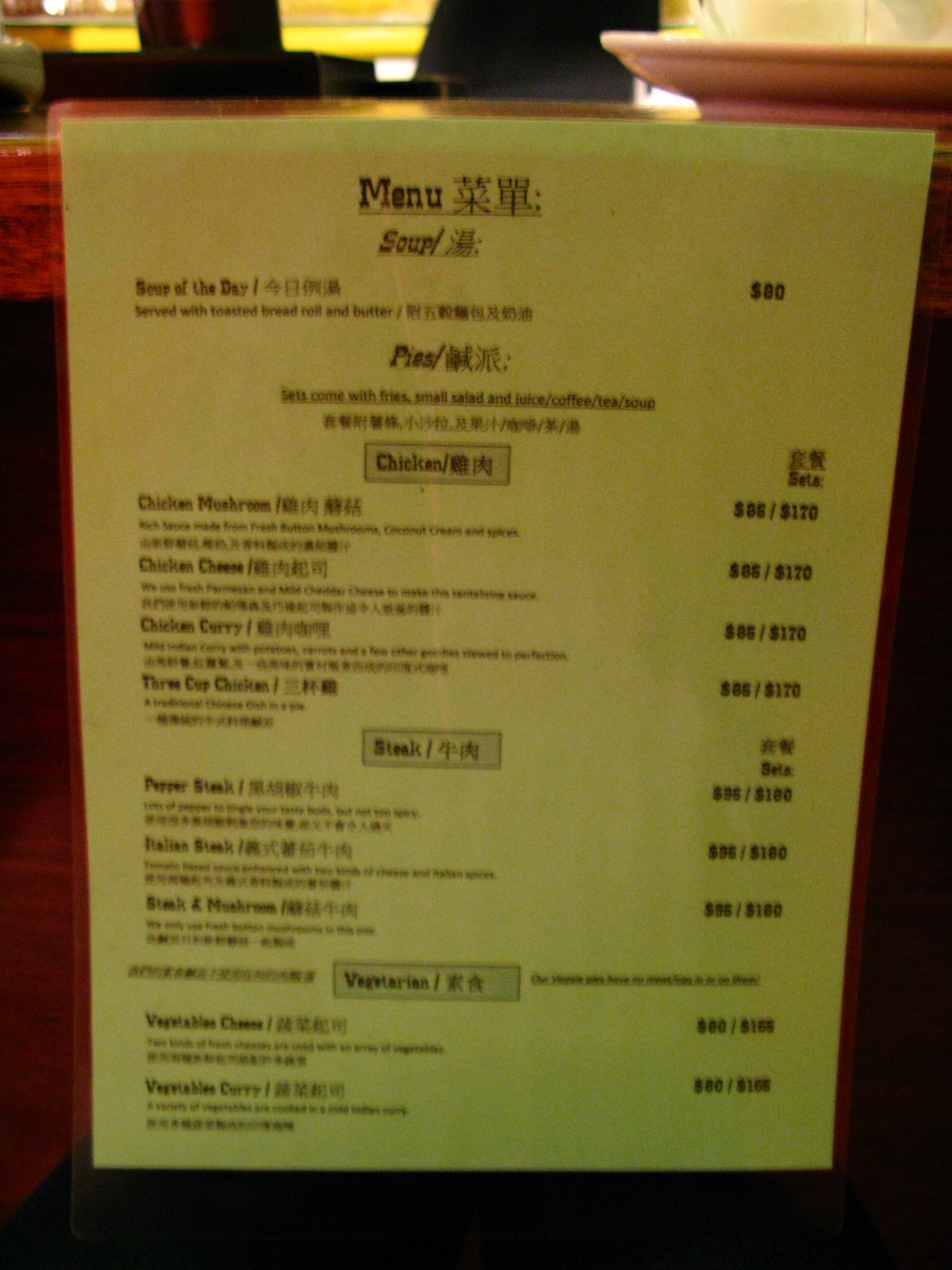The image depicts a menu card featuring both English descriptions and corresponding Chinese characters for each item. The menu appears to be laminated and is positioned upright, possibly on a table against a wall.

At the top, the word "Menu" is prominently displayed, followed by a section labeled "Soup / 汤" with an exclamation point. The first item listed is "Soup of the Day," served with a toasted bread roll and butter, priced at $80 (likely in a currency other than USD). 

Below the soup section, there's a heading "Pies / 馅饼." This section is detailed with options that include a side of fries, a small salad, and a choice of juice, coffee, tea, or soup. The pies are categorized under three banners:

1. **Chicken Pies / 鸡肉馅饼**
    - Chicken Mushroom
    - Chicken Cheese
    - Chicken Curry
    - Three Cup Chicken

2. **Steak Pies / 牛排馅饼**
    - Pepper Steak
    - Italian Steak
    - Steak and Mushroom

3. **Vegetarian Pies / 素食馅饼**
    - Vegetables Cheese
    - Vegetables Curry

Each section is illustrated with care, ensuring clear distinction between the varieties. The meticulous layout and bilingual descriptions make the menu accessible to both English-speaking and Chinese-speaking patrons.